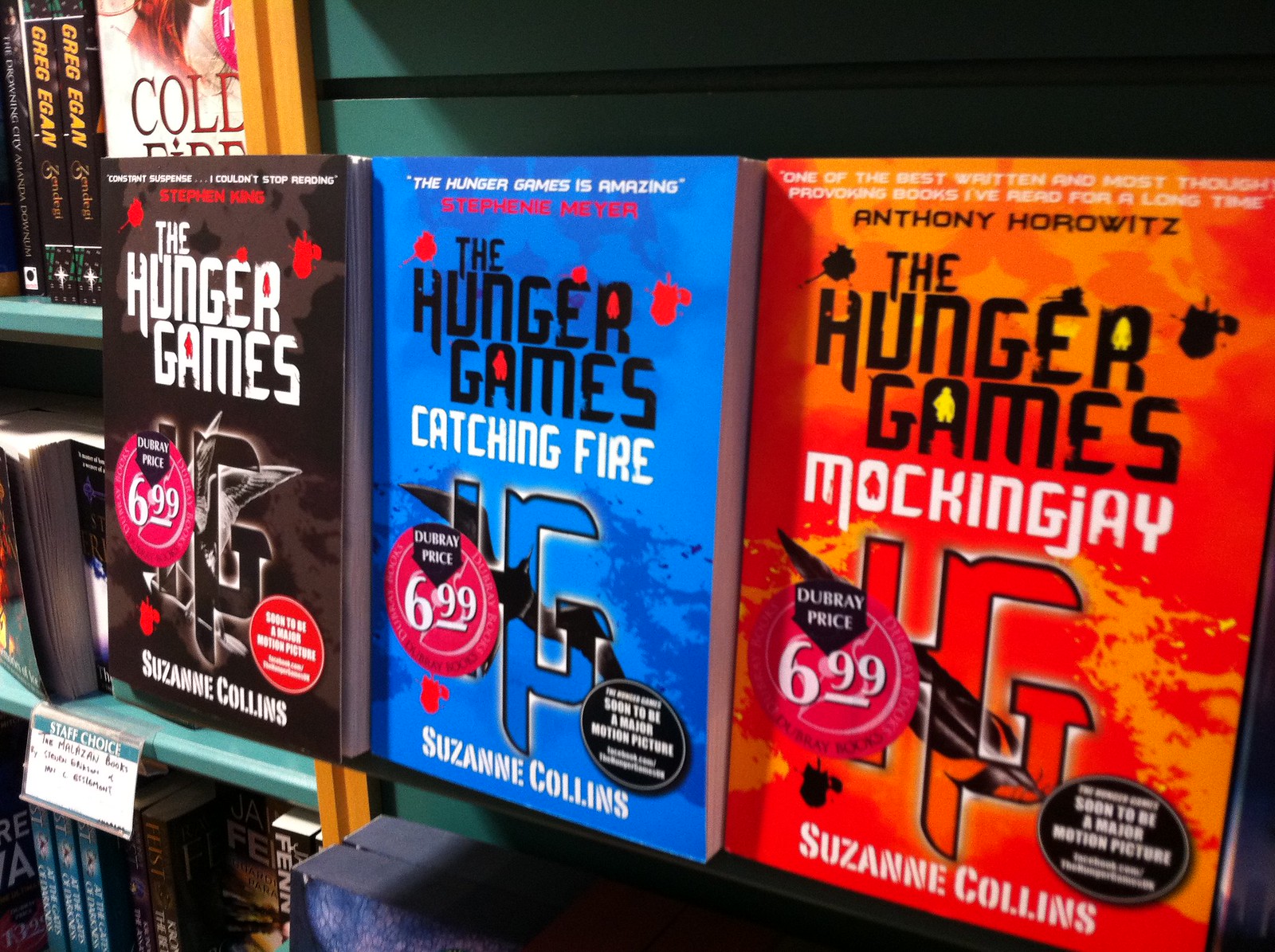The image appears to be taken indoors at a bookstore and focuses on three differently-colored editions of "The Hunger Games" series by Suzanne Collins. The first book, "The Hunger Games," has a black cover adorned with red blood specks, featuring the title in white and a price tag of £6.99. The second book, "Catching Fire," sports a blue cover with similar red blood specks, with "The Hunger Games" in black and "Catching Fire" in white, also priced at £6.99. The third book, "Mockingjay," comes in an orange cover with black blood specks and has "The Hunger Games" in black and "Mockingjay" in white, similarly priced at £6.99. Additionally, the black book features a red circle in the bottom right corner, and there are endorsements on the books from well-known authors. The background reveals a bookshelf on the left with three shelves containing various books, including works by Greg Egan and a title that says "Cold Fire." Other books are also present on a staff choice shelf.